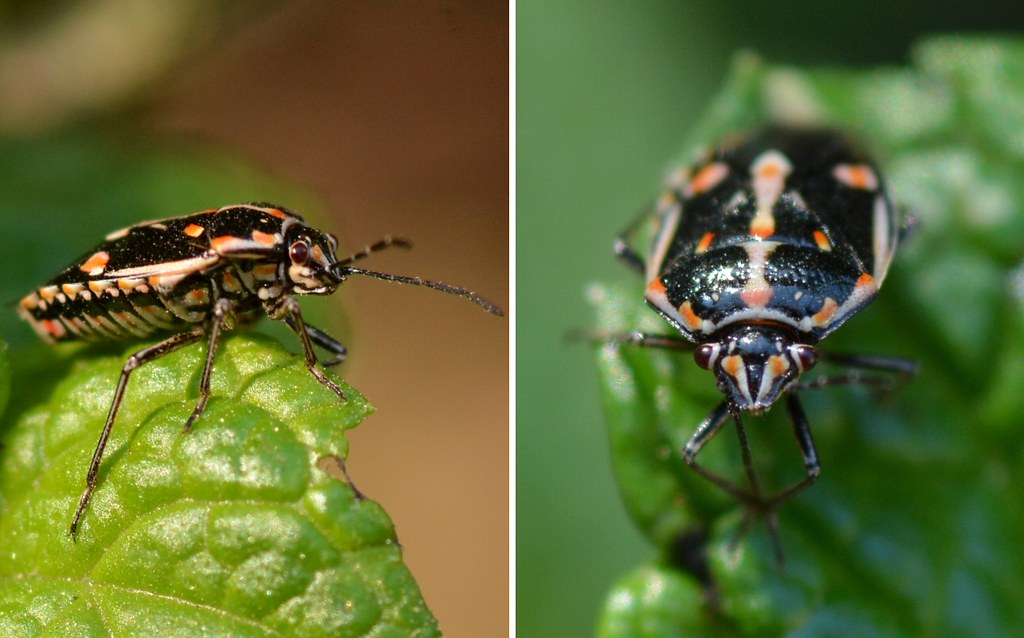The image is a collage of two photographs showcasing the same species of beetle, arranged within a rectangular frame. A thin white border encircles the perimeter and splits the image down the middle, dividing it into two equal halves. Both photographs are also rectangular, oriented such that their heights are twice their widths.

In the left photograph, the beetle is depicted in profile, facing right. It rests on a large, leafy green plant, which appears to have been partially devoured, with visible bite marks. The beetle itself has a predominantly black shell adorned with distinct orange spots and accented with white lines along its edges.

The right photograph provides a front-facing view of the beetle, capturing it as if it’s peering directly into the camera. The beetle’s head has a triangular shape, with pronounced brown eyes encircled by white rings. Two orange-centered white triangles point down towards its nose area. Its shell mirrors the pattern seen in the first image, featuring a black base with a central line of white and orange dots and additional orange spots scattered near its top-left, bottom-left, and bottom-right corners.

Both photographs share a common background— a light green, blurry environment that emphasizes the beetle and the large leaf it’s on, highlighting the intricate details and coloration of this fascinating insect.